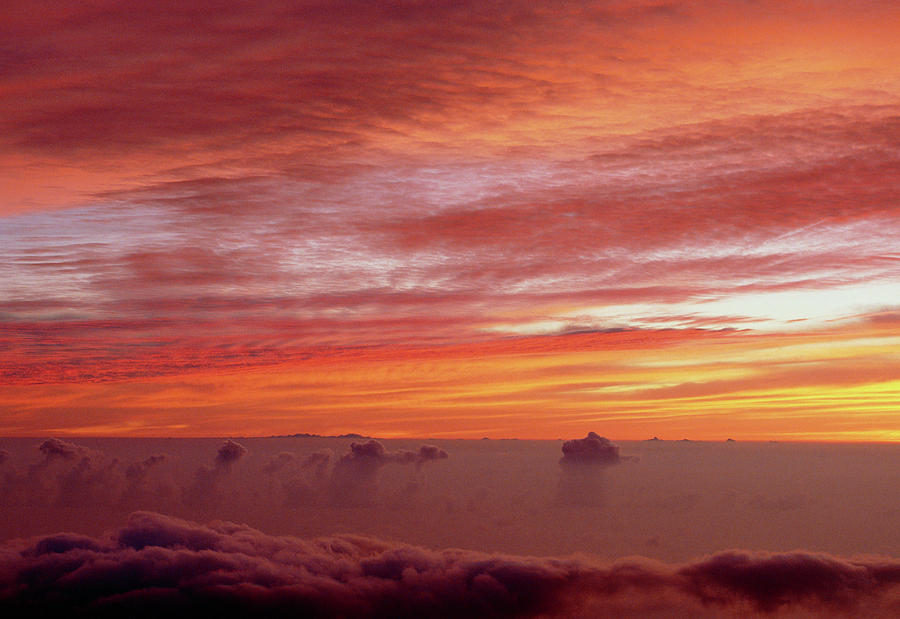This detailed photograph captures a serene sunset, as observed from a high vantage point, possibly an airplane. The sky is painted with a gradient of muted yet rich colors, featuring shades of orange, purple, dark red, and hints of yellow, giving a peaceful, almost ethereal vibe to the entire scene. In the foreground, fluffy, soft-looking clouds, that resemble feathery lumps, float, while a solid strip further back sparks curiosity—it could be another bank of clouds, a distant horizon or even a lake, adding a layer of mystery to the image. Beyond this, the horizon bathes in the beautiful warm colors of the setting sun, with patches of white and the occasional appearance of blue sky peeking through, all indicative of high-altitude cirrus clouds breaking up slightly. The entire photo wonderfully captures the serene beauty of the sky during sunset, with no identifiable landmarks or elements, emphasizing the timeless and universal beauty of nature on display.